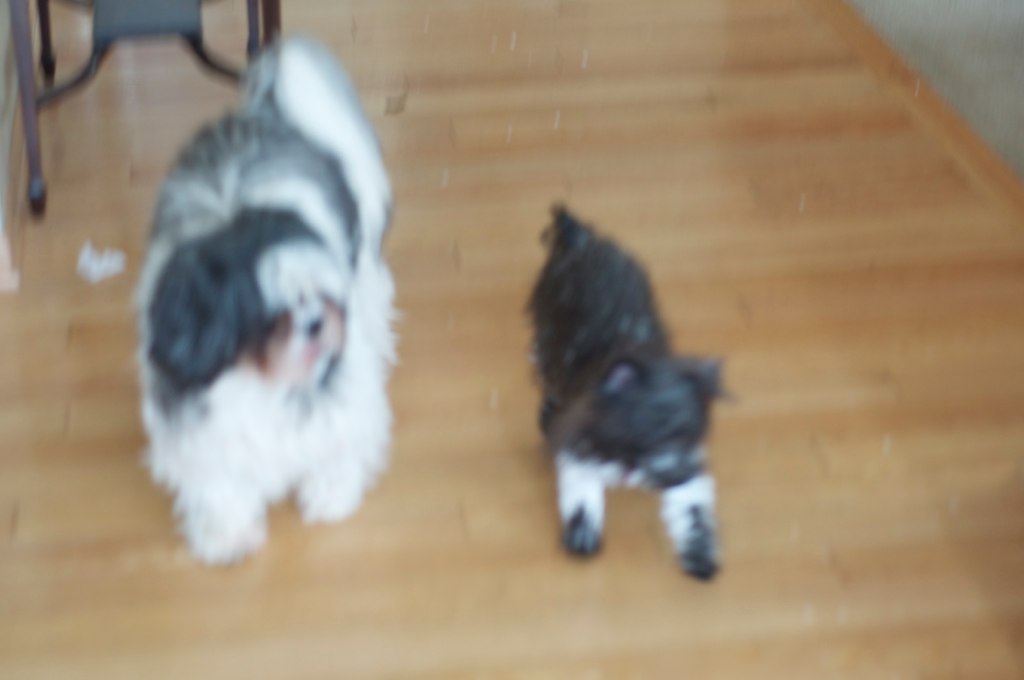In the image, we observe a slightly blurred scene of two dogs indoors on a brown hardwood floor. The dog on the left, viewed from the front, is predominantly white with a black head and patches of gray along its body. It is lying down comfortably. To the right is a smaller black dog, distinguishable by its white front paws that have black tips. The remainder of this dog's body is black. In the top left corner, partially cut off, there is an outline of a chair's lower half. In front of the chair lies what appears to be a crumpled white object. The top right corner of the image features a faint gray background, but the main focus remains on the dogs and the brown floor.